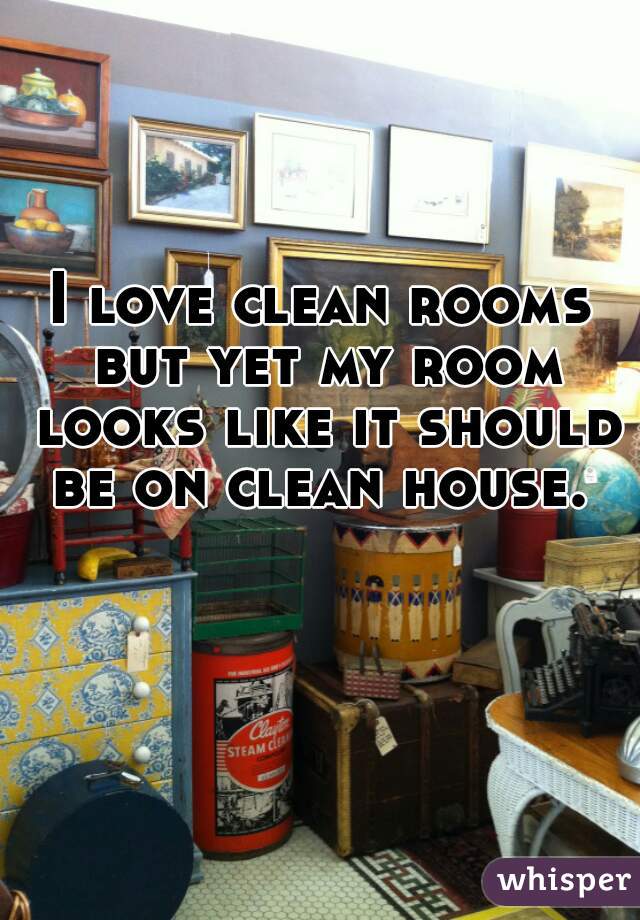This image depicts a cluttered room that could be part of an office, garage, or perhaps a booth at a flea market, filled with various vintage items and furniture. There is an assortment of pictures, both large and small, covering the blue walls with brown trim. The pictures are framed in different styles, including brown, silver, and gold. Centrally mounted over the pictures is a bold statement in black letters, outlined in white, reading, "I love clean rooms, but yet my room looks like it should be on Clean House," spread over four lines. Below the pictures, a large canister resembling a banjo drum is situated atop a brown chest. To the right of this setup stands a tall cylindrical container in black, red, and white. An old dresser with gray and yellow drawers fitted with white knobs is positioned to the left. On the far right, there's a white wicker table with a brown top, housing an old black typewriter and other miscellaneous objects. A large blue globe is partially visible in the background on the right side of the image. The bottom right corner features the word "WHISPER" highlighted in purple letters. The scene is chaotic and packed with various antiques and furniture, contributing to its overall disordered yet intriguing atmosphere.